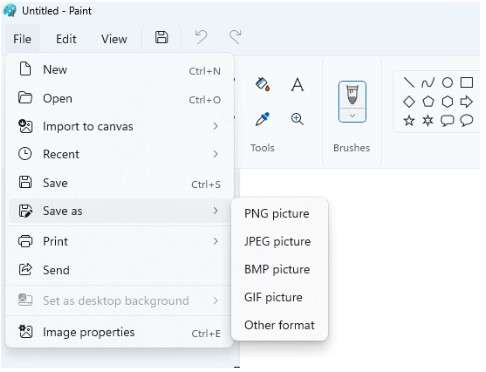In this detailed screenshot, the interface of a paint application is prominently displayed with various sections and options clearly visible. The title bar at the top left corner reads "Untitled - Paint." Below the title bar, the menu options are laid out horizontally from left to right: "File" (which is currently selected), "Edit," "View," a print icon, and two arrows for navigation.

Within the expanded "File" tab, a list of categories is presented vertically in the following order: "New," "Open," "Import to Canvas," "Recent," "Save," "Save As," "Print," "Send," "Set as Desktop Background," and "Image Properties." Adjacent to these categories are options for saving files in different formats: "PNG picture," "JPEG picture," "BMP picture," "GIF picture," and "Other format."

To the right of these file format options is the "Tools" section, featuring four distinct icons. Moving further right, the "Brushes" section is visible, followed by an array of 12 tool icons set against a light gray background. Both the left and top parts of this section have a similarly light gray background.

Concluding the interface overview, the very bottom right section of the screen has a white background, providing a clean and clear space in the interface layout. This comprehensive layout visualization offers a thorough representation of the paint application's user interface.